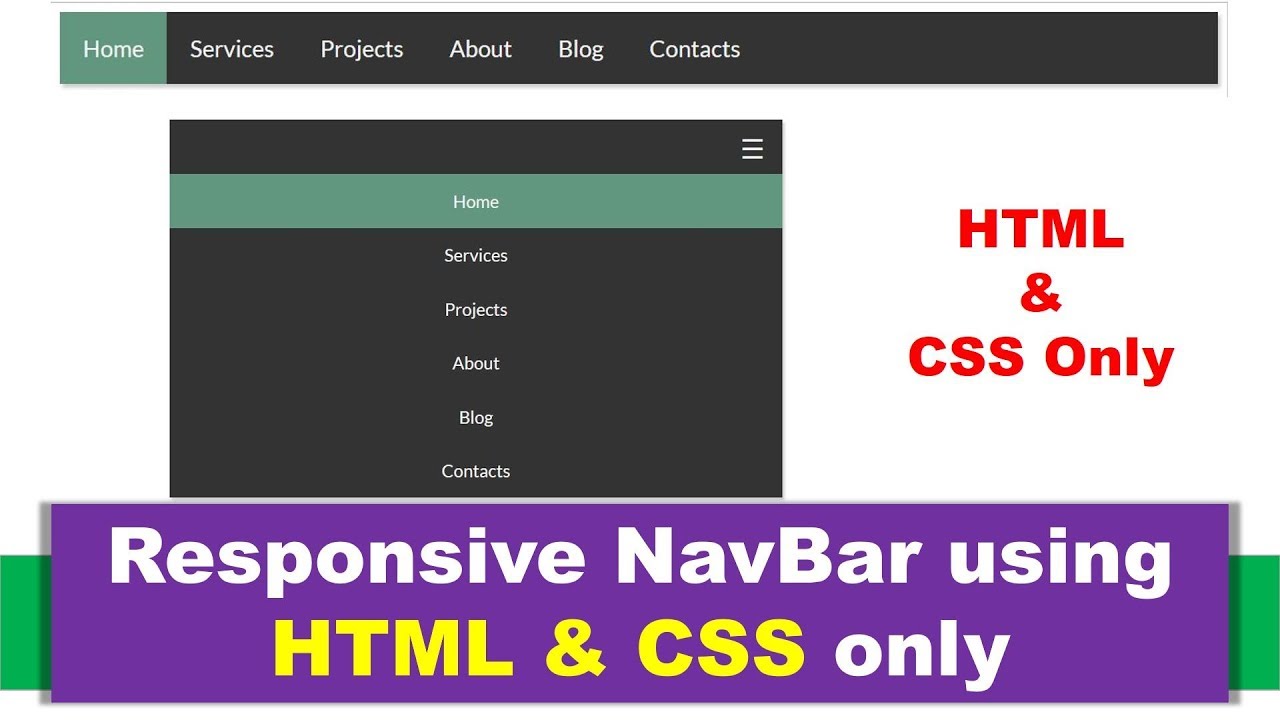The image depicts a web page with a clean, predominantly white background. At the very top of the page, there's a black horizontal border extending across the width of the page, which includes a subtle green background on the left side. The word "Home" is set against this green background in white text, while the other menu items— "Services," "Projects," "About," "Blog," and "Contact"— are displayed in white text against the black background, making "Home" prominently highlighted.

Below this top section, aligned towards the left side, is a rectangular box with a black background. In the top right corner of this box are three horizontal white lines, resembling a menu icon. Directly underneath, a green strip displays the word "Home" in white text, once again highlighted. The rest of the items within this box— "Services," "Projects," "About," "Blog," and "Contacts"— are in white text against a black background. To the right of this box, the phrase "HTML and CSS only" is presented in red text.

At the very bottom of the page, a purple banner is notable for containing the phrase "Responsive Navbar Using." This is rendered in white text. Following this, the phrase "HTML and CSS" appears in yellow text, and the final word "only" is in white text, all against the same purple background. This purple banner is superimposed over a green border, with the green edges visible on the left and right sides of the banner.